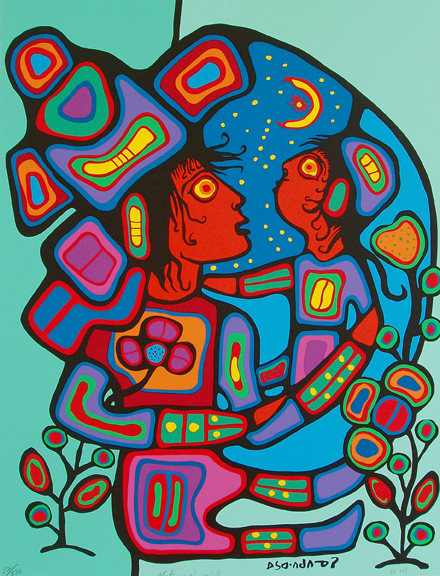The image showcases a vibrant and highly stylized abstract painting with a light greenish to aquamarine background that darkens on the left side and lightens on the right two-thirds. Dominating the composition are two figures rendered with an intricate blend of shapes and colors. The larger figure, positioned seated with legs extending to the right, faces forward with its head turned to the right, and the smaller figure, appearing to be a child, is oriented towards the larger figure with an arm reaching out towards its neck. Both figures have red faces, black spider-webby hair, and striking yellow eyes with black outlines. The larger figure features a flower emblem on its chest and ornate designs on its limbs, while the smaller one wears a colorful cap adorned with blue, purple, pink, green, red, and yellow strands.

Above the figures, a crescent moon with yellow stars and a red and yellow sun inside is prominently displayed in a blue sky. Surrounding the figures are multicolored flowers, characterized by oblong and circular leaves with black outlines. These flowers appear behind the larger figure on the left and the smaller figure to the right. The bottom right corner of the image bears an unreadable signature, ending with a sideways 'P' and a question mark. The overall impression evokes a blend of Aztec influences and modern abstract art, with a rich, blocky stylization that gives the figures a somewhat surreal, almost zombie-like appearance.